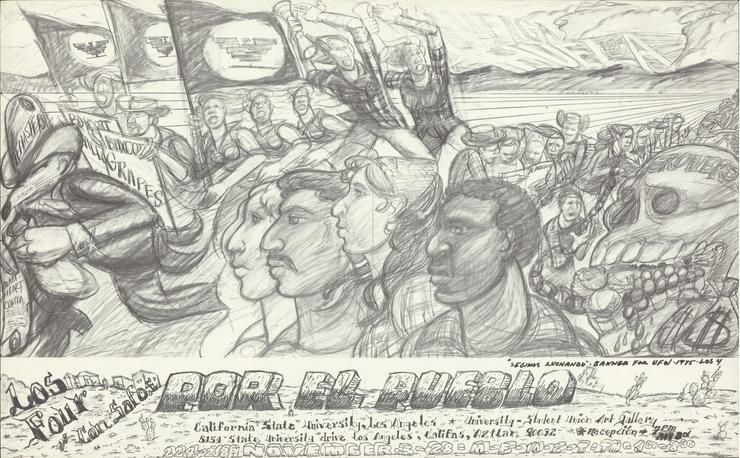This image is a detailed pencil sketch on cream-colored paper. The entire background is cream-colored, and the drawing depicts a demonstrative scene. At the bottom of the sketch is a hilly landscape with cacti growing in front, where the words "Los 4 Con Safos" and "Por el Pueblo" are inscribed. To the left side of this area, small buildings are visible. Along the bottom, there is also some small text that appears to reference "California State University, Los Angeles," "University Student Union Art Gallery," and a date that looks like "November 3, 28."

The main part of the image shows a group of people at a protest or demonstration, some holding flags and signs with messages like "boycott grapes." Notably, there are four larger faces in the forefront—two men and two women—depicting different ethnicities. Additionally, flags with bird emblems are highlighted. Among the group, on the far left, is a rat-like figure in a suit and a cowboy hat labeled "Teamsters," holding a large bag of money, appearing to run away.

Towards the right side of the image, a grotesque skeleton with the word "Grovers" on it is illustrated, adorned with money bags and jewelry spilling out of its teeth. This skeleton seems to represent a malevolent entity surrounded by people. Above the primary scene, the sky has rolling clouds and hills, adding depth to the backdrop. Overall, it portrays a powerful narrative of resistance and protest within a community.